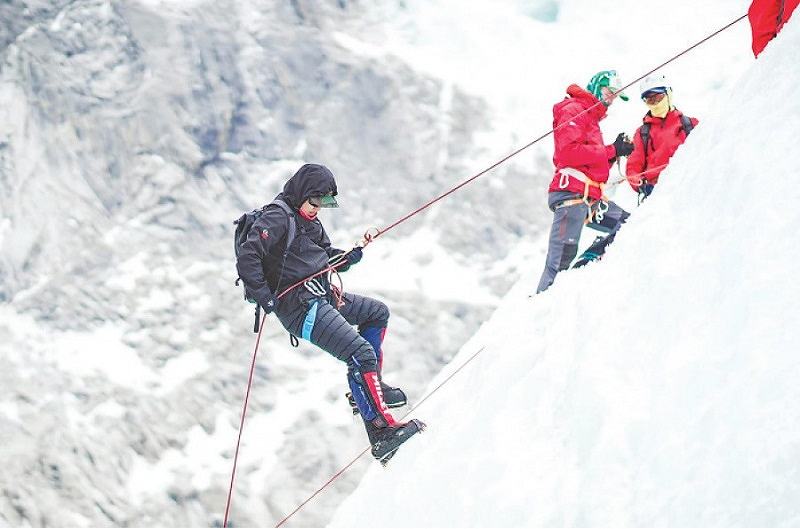This horizontally aligned rectangular photograph captures a dramatic moment of mountain climbing in a snowy landscape. In the foreground, a man clad in a black hooded jacket, striped pants, and possibly wearing ice climbing boots with picks, is meticulously climbing a steep, snow-covered slope. He has a green baseball cap peeking from under his hood and is wearing sunglasses. His intense focus is directed downward towards his hands gripping a red rope tethered around his waist, hinting at the difficulty of the climb. The snowy slope he's on dominates the right side of the image.

To his left, two other men are slightly higher up the slope. Both are wearing red jackets; one has a green hat and gray pants, while the other has a blue hat and stands out in the stark wintry backdrop. They appear to be conversing but are clearly part of the climbing expedition. In the background, on the left side of the image, a monumental gray cliff rises in the distance with patches of white snow clinging to its jagged surface. The overall scene evokes a sense of camaraderie and the grim challenge posed by winter mountain climbing.